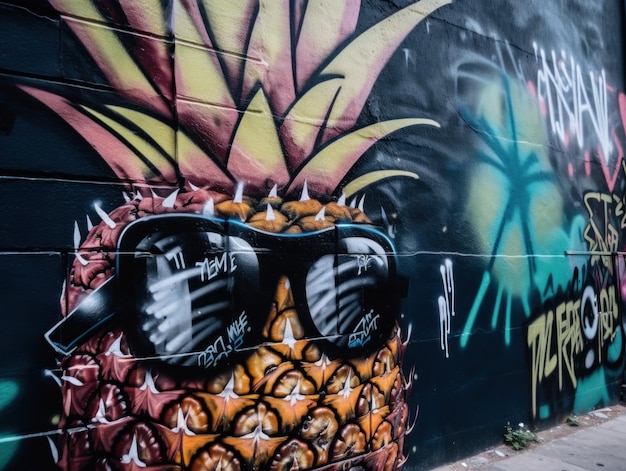The image features a striking painted mural on a black concrete block wall in a city. Dominating the left side of the mural is a large and vibrant pineapple, adorned with huge black sunglasses that occupy more than half its face. The pineapple's exterior is tinged with a bright pink hue, transitioning into a traditional golden color as it ripens. Its leaf crown, painted in playful shades of pink and yellow, extends energetically from the top. The sunglasses reflect stylized, non-English graffiti lettering, adding an intriguing layer of interaction within the artwork. 

To the right of the pineapple, the wall transitions into a cyan blue splash with intricate lines, shifting away from the predominantly black background. Further right, a section of the wall displays a neon light pink area with more letters, although the distance and angle render them illegible. Beneath this, beige letters spell out yet more indecipherable text. Additional illustrations, including a beigish circular design intersected by bluish lines and another star-like drawing, contribute to the mural's dynamic and colorful composition, blending bright blues, whites, golds, and more black, all accented with pink outlines.